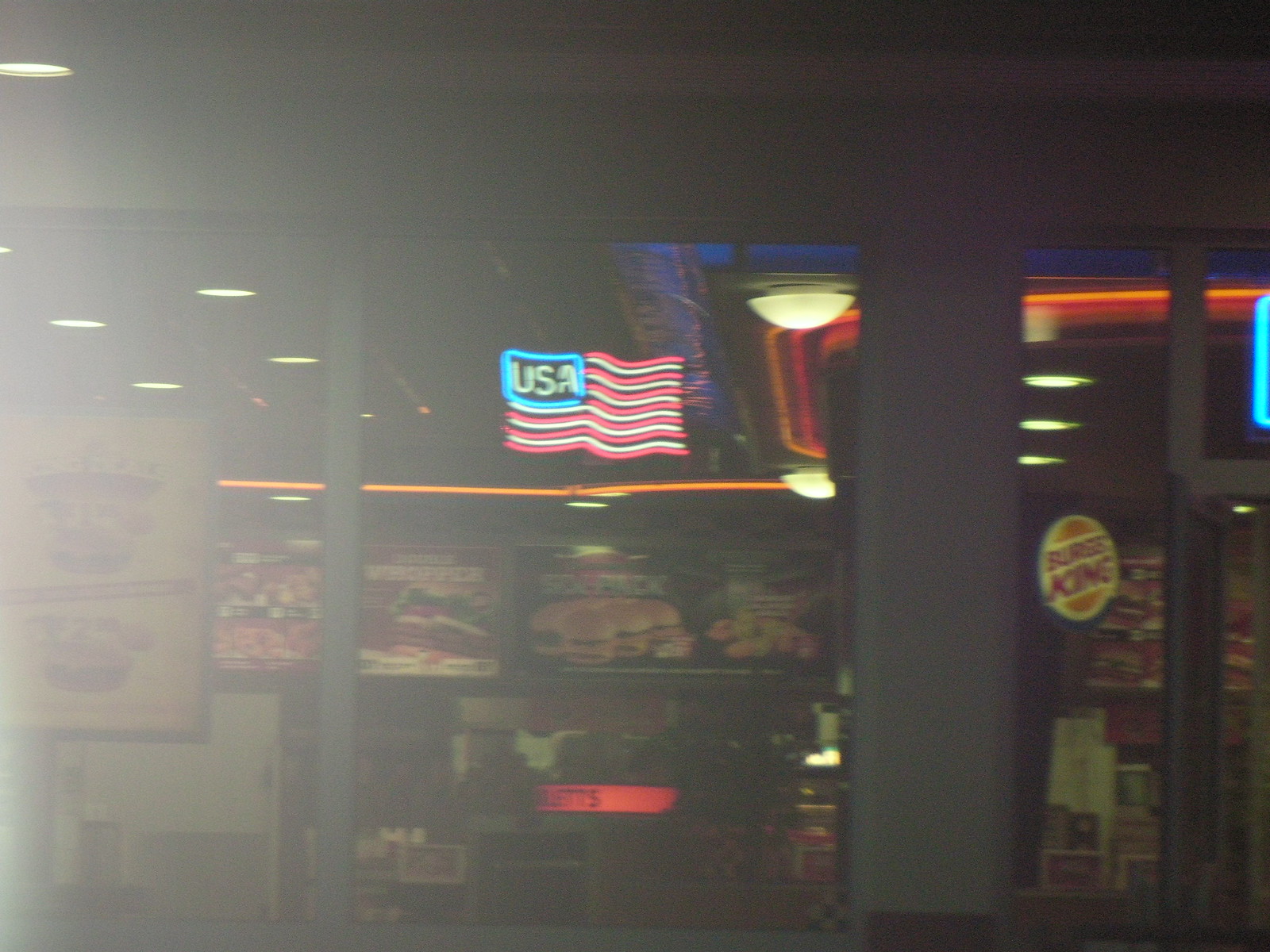This photograph appears to be taken from outside a fast food restaurant during nighttime. The image is slightly blurred, but several elements are distinguishable. The establishment is identified as Burger King, evident from the recognizable emblem visible through the glass windows. A striking neon United States flag adds a touch of illuminated patriotism to the scene, likely affixed to the interior side of the window. The building's exterior features glass walls framed by sturdy black pillars or supports. Inside, though the details are hazy, we can discern various signs and menus on the walls. Blurry images of signature items such as the Whopper and other hamburgers, along with some menu boards, are faintly visible, hinting at the offerings of this well-known fast food chain.